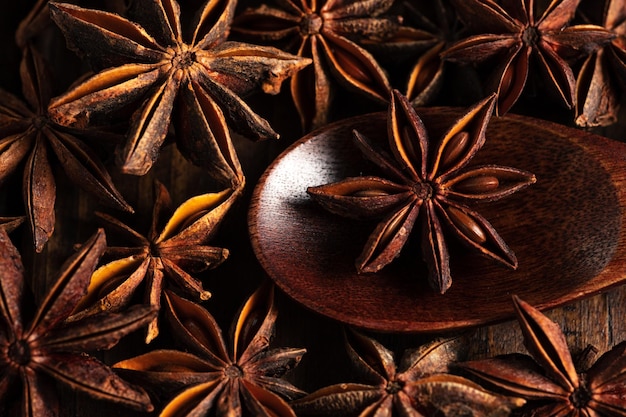In this close-up photograph, a collection of star anise spices is displayed on a dark brown, wooden surface. The star anises, which resemble dried, star-shaped flowers with brown seeds nestled inside their arms, are scattered across the image. The photograph prominently features a wooden spoon positioned on the center right, showcasing its main, wider part only. One star anise rests on top of this brown spoon, while the rest are strewn across the table. The intricate details of the star anise pods are clearly visible, highlighting their unique structure and rich, earthy tones.